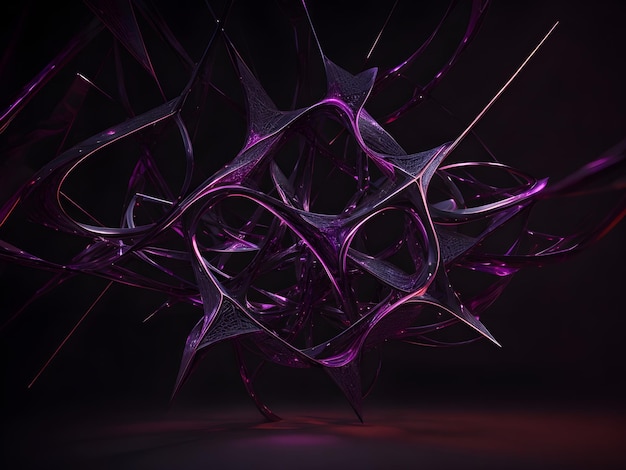This image depicts a digital artwork featuring an intricate, iridescent purple splash set against a predominantly black background, giving it an outer space-like appearance. The background is dark, with slight purple and maroon shading at the bottom, creating the illusion of a celestial sphere. The splash itself is a high-definition, abstract design with multiple spikes and fluid, undulating forms, reminiscent of non-Euclidean fluid dynamics, similar to cornstarch and water vibrations on a speaker. It has a complex three-dimensional effect, with varying shades of purple and prominent white highlights. Within the abstract shape, there are four large circular forms and multiple long, skinny projections, creating a sense of depth and intricate detail in the artwork.